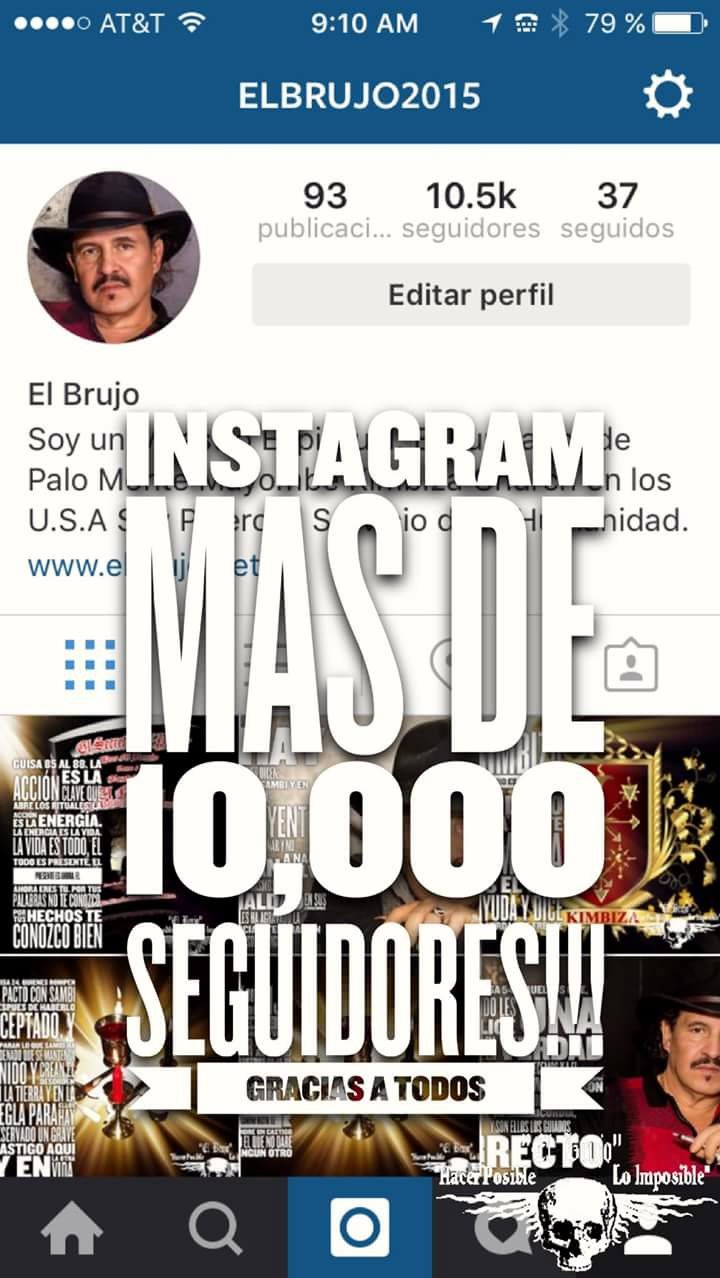This is a portrait-style image of a vintage Instagram screenshot featuring the old Instagram layout. The interface includes a large grey bar at the bottom with home, search, camera, heart, and profile icons. The profile icon is highlighted in black, indicating the user is currently on their personal profile page. The account belongs to "Elbrujo2015," who has 10.5k followers and is following 37 accounts. The interface is entirely in Spanish, with "editar perfil" written in bold white letters and a message that reads "Instagram, mas de 10k seguidores, gracias a todos," which translates to "more than 10k followers, thank you all." The profile picture is of a Mexican man approximately 40 years old, with a square face, thin mustache, thin soul patch, dark black cowboy hat, and longish brown hair. His username and various details are shown at the top, with some clutter due to white text, making it challenging to read. There are no visible advertisements for upcoming shows, but the layout and symbols at the bottom such as a house, magnifying glass, and camera button are clearly visible, indicating the app is Instagram.